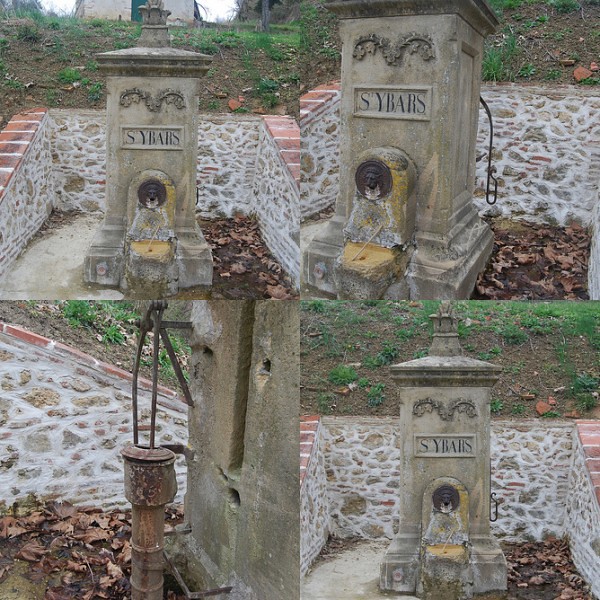The image is a collage of four square photographs, each showcasing different angles of a small, ornate concrete column, which appears to be a historical or decorative monument. This monument stands about six to eight feet tall and features a distinct cornice at the top. The front of the column prominently displays a label that reads "CYBARS" or "SYBARS," and below the label is a circular plaque with the image of a lion's head, possibly indicating that it once functioned as a water fountain. The lower left image in the collage reveals the back of the column, highlighting exposed metallic attachments and a possible pump mechanism. Surrounding the column is a recessed alcove built into a small, grassy hill with exposed soil. Above this alcove, partially visible, is a building, indicating the column's location at the base of an incline. The environment is accentuated by a rock wall and scattered leaves, adding to the aged and historical feel of the site.